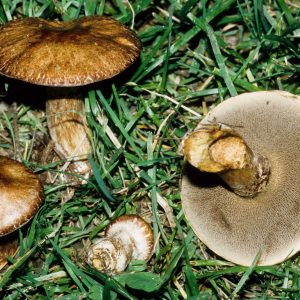In the close-up photograph, a cluster of four brown mushrooms grows amidst a lush patch of green grass. Dominating the top left is a mature mushroom, with its dark brown cap extending from a sturdy stem. Beneath it, only a portion of another cap is visible, hinting at another mushroom. Centered towards the middle and to the right, two mushrooms have toppled over, their stems pointing upwards. One of them, a large mushroom, lies on its side, revealing its lighter, spongy underbelly with a slight whitish fuzz texture. Near it is the smallest mushroom, almost white beneath its brown top, also knocked over and displaying its underside. These mushrooms, varying in size and orientation, cover approximately 75% of the image.